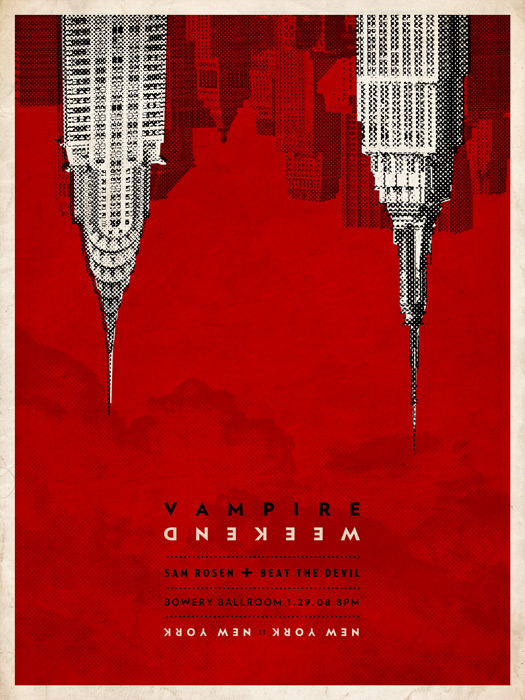This poster, designed in portrait mode with light tan marbled borders, vividly advertises a performance gig with a striking depiction of the New York City skyline. The entire image is dominated by a rich red background, complemented by black windows and clouds. The skyline, including the iconic Empire State Building, is inverted, positioned at the top of the poster, creating a dramatic effect reminiscent of fangs. In bold black text, the word "Vampire" captures immediate attention, followed by the word "Weekend" written upside down and backward in white print. Below these, a row of dotted lines separates the performers' names: "Sam Rosen plus Beat the Devil." Further down, more dotted lines precede the venue details: "Bowery Ballroom, 1.29.08, 8 PM." At the very bottom of the poster, another row of dotted lines frames the final inverted text, "New York, New York," enhancing the overall surreal and creative design.